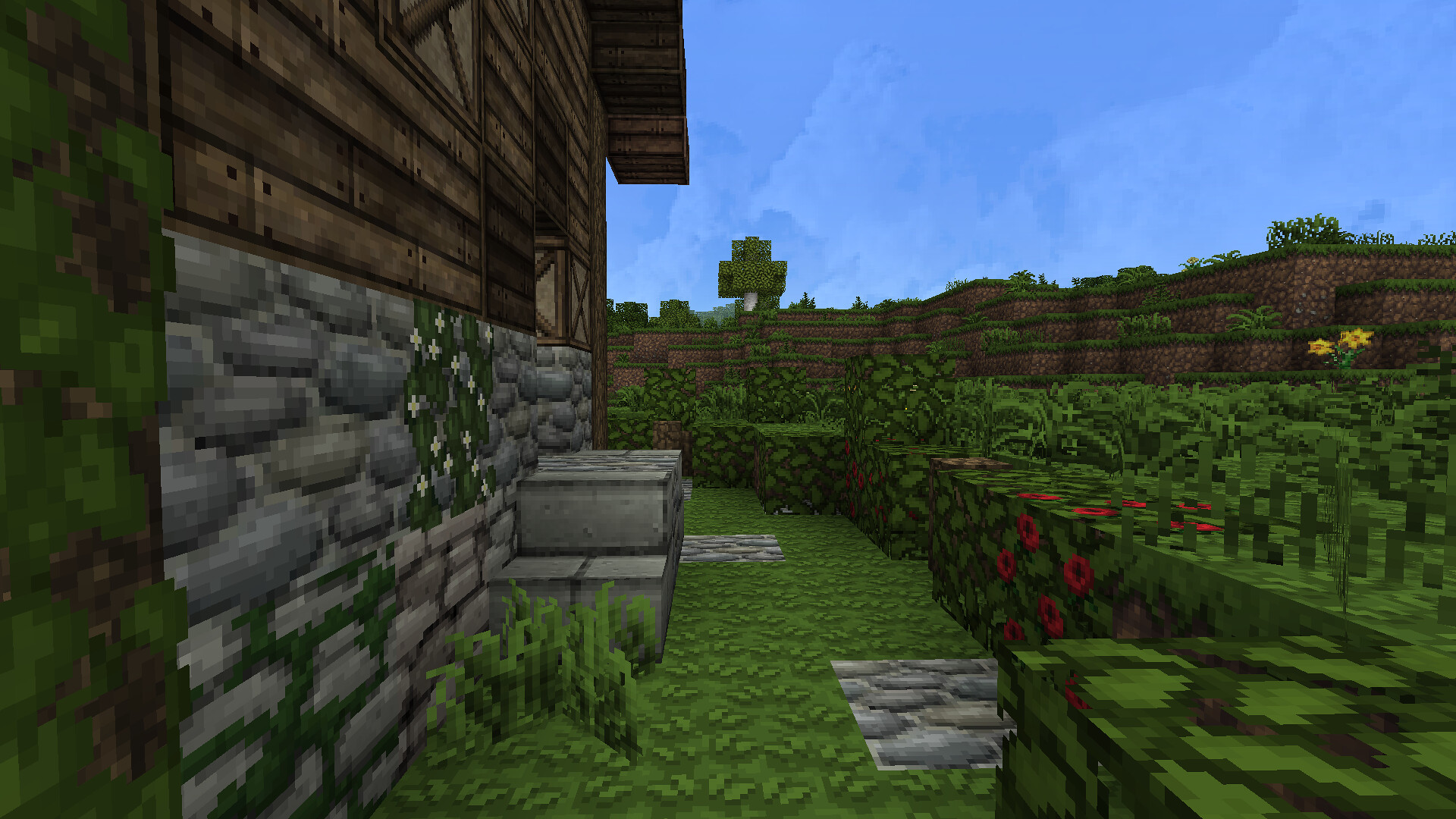This 16:9 resolution screenshot from the video game Minecraft features an unmistakably pixelated and blocky aesthetic. Dominating the left half of the image is a structure that resembles a cabin or country cottage. The lower portion of this building showcases a detailed cobblestone texture interspersed with accents of ivy and white flowers, lending a rustic charm. Rising above, the upper half of the building is crafted from dark wooden planks, amplifying the appearance of a classic wooden cabin.

Adjacent to the building, a manicured lawn is visible, featuring dark stone stepping stones and a neatly arranged hedge adorned with red flowers. This lush, green expanse extends to the right half of the image, where dense vegetation, including additional bushes and yellow flowers, can be seen.

In the far background, the landscape shifts into terraced cliffs, characterized by brown, dirt-patterned blocks that step unevenly upward, each tier topped with a patch of green grass. Hovering above this scene is a clear blue sky, completing the picturesque setting devoid of any text or overlay. Every element within this image is constructed from simple, textured blocks, maintaining Minecraft’s signature blocky style without any round edges.